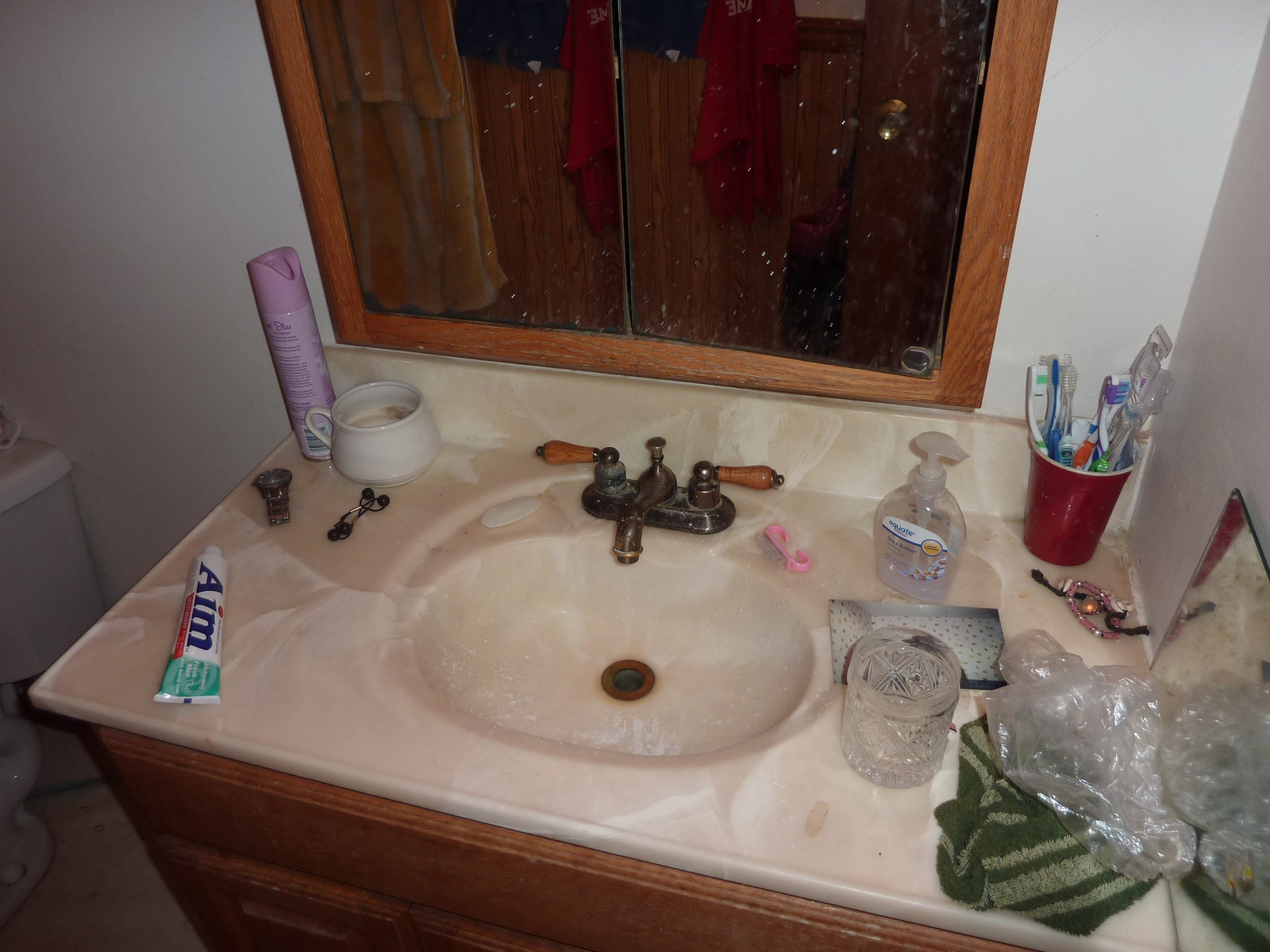In this image of a cluttered bathroom, the walls are predominantly white with sections of wood paneling. A large, dirty mirror with a brown frame and potential sliding doors is mounted on one wall. The mirror barely reflects a wooden door with a brass handle, alongside a red or burgundy shirt with yellow writing hanging on the door. Also visible in the reflection is a yellow and white towel.

The bathroom counter has a wood-colored base topped with a faux quartz or granite surface, which extends to the sink basin made of the same material. The sink features a bronze-colored faucet with wooden handles. Various items clutter the countertop, including a can of air freshener, a wristwatch, a hairband, a cup of coffee, AIM toothpaste, a crystal cup, liquid soap, a red Solo cup filled with multiple toothbrushes, and a friendship band. Additionally, a plastic bag and a dark and light green washcloth are also present.